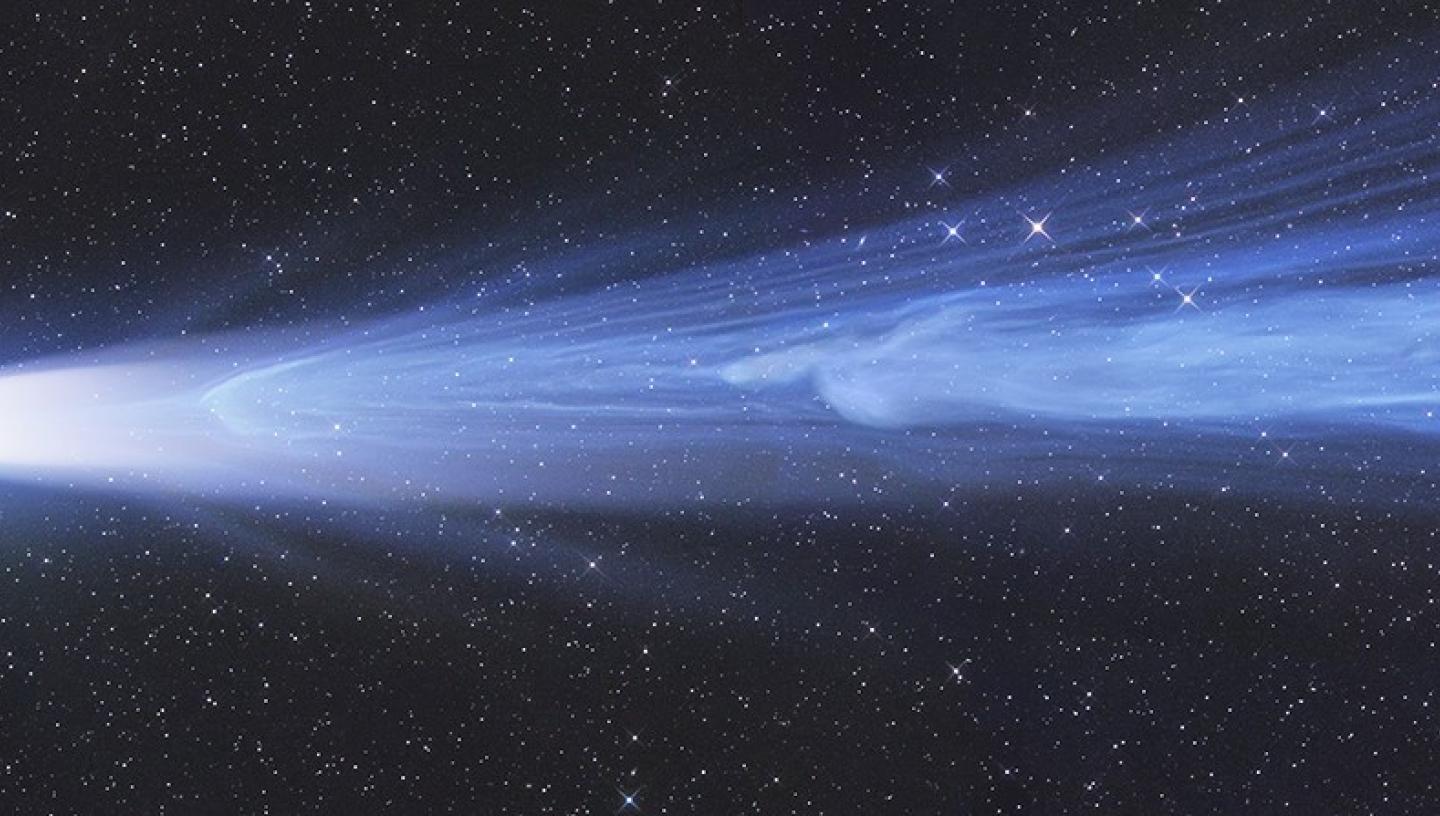The image is a detailed illustration of outer space featuring a predominantly black background scattered with numerous white speckles representing stars and galaxies. The primary focus of the image is a prominent streak of light that resembles a comet's tail or a bluish fog. This streak travels from the right side of the image to the left, growing dimmer and wider as it progresses. Towards the left side, the light intensifies, becoming remarkably bright. The streak of light exhibits a wavy pattern and is set against a stunning backdrop of countless stars, creating a vivid and dynamic impression. The image, likely computer-generated or an artistic illustration, evokes a sense of space travel or a cosmic event, suggesting a scene that could be right out of a sci-fi movie.